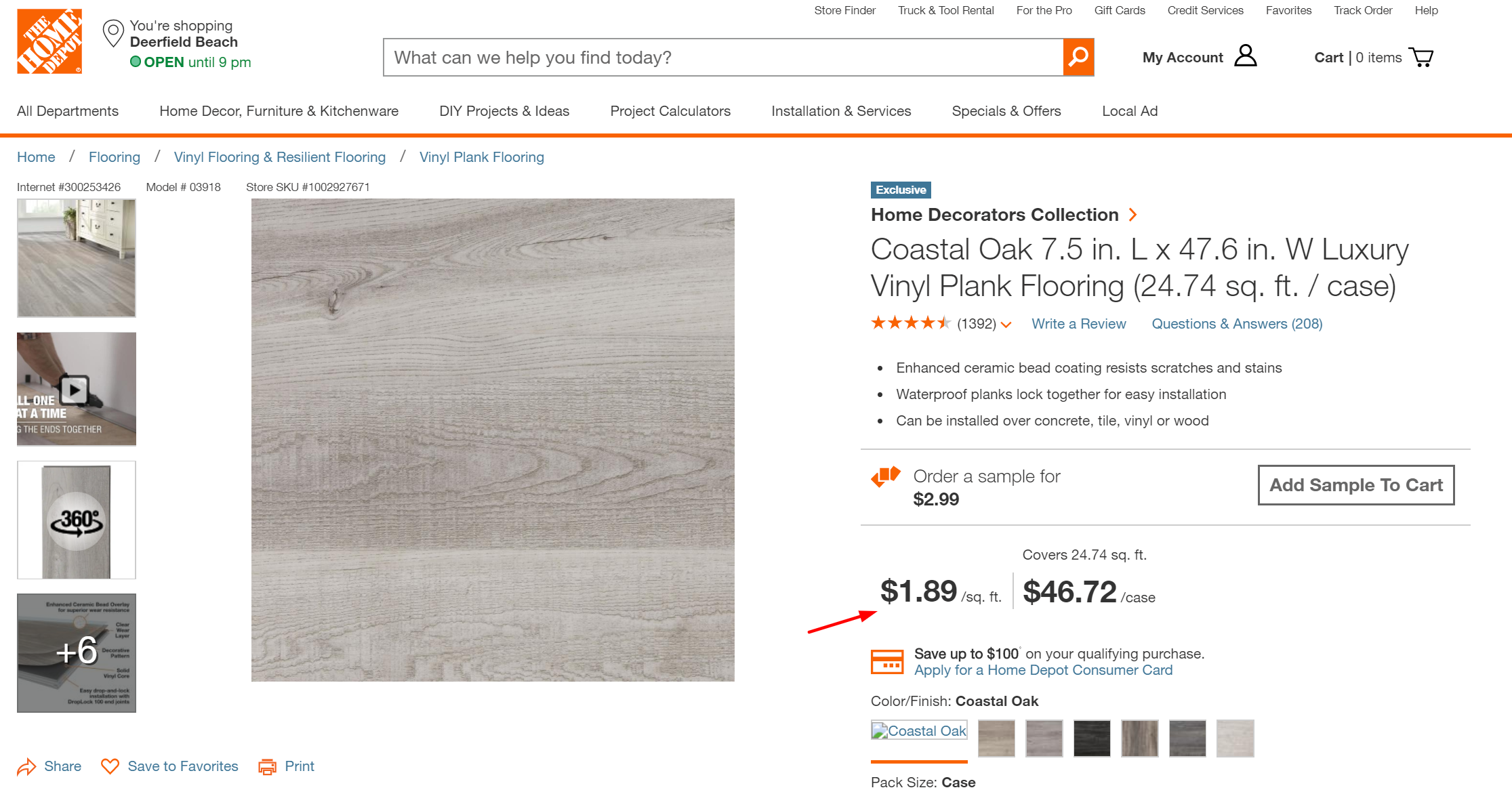This is a screenshot of the Home Depot website. In the top left corner, the recognizable orange and white square Home Depot logo is displayed prominently. At the center of the header, there is a search bar with the prompt, "What can we help you with today?" and an orange search icon that complements the Home Depot brand colors. 

To the right of the search bar, there are options to access your account and view your shopping cart for adding items. The website indicates the nearest store location as "Deerfield Beach," which is noted to be open until 9 p.m. 

The navigation menu is robust, featuring categories such as "Old Apartments," "Home Décor," "Furniture and Kitchenware," "DIY Projects and Ideas," "Project Calculators," "Installation Services," and "Specials and Offers." Additionally, there is a "Local Aid" section for community support resources.

A prominent product advertisement occupies the main body of the webpage. It showcases a luxury vinyl plank flooring option named "Coastal Oak," measuring 7.5 inches wide from the Home Decorators Collection. The flooring is priced at $1.89 per square foot, with a red arrow emphasizing this price point. For reference, a single case covers 24.74 square feet and costs $46.72. An offer is highlighted below the pricing, mentioning savings of up to $100 on qualifying purchases when applying for a Home Depot credit card. The product is available in multiple colors, and additional visual aids include a layout video along the left-hand side to help customers visualize the product in use.